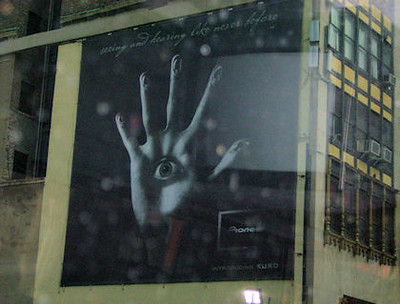In the photograph, a striking billboard dominates the side of a large building. The advertisement features a black background with a central focus on an eerie hand. The hand is depicted with fingers spread wide apart, each fingertip adorned with an eyeball, including a prominent eyeball in the palm, all staring straight ahead. Positioned at the top of the billboard in a white, cursive font is some text, though it is difficult to decipher. The brand's logo, possibly reading "Prone" or something similar, is located in the lower right-hand corner of the ad. The building itself has numerous windows, framed by yellow panels, and several windows are outfitted with air conditioning units. Overall, the image presents a juxtaposition between the ordinary urban façade and the unsettling, artistic billboard.